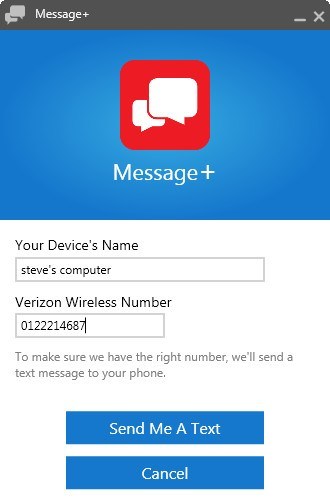This image features a screenshot of a verification screen for the Message+ application. At the top, there is a black bar with two small white icons resembling quote boxes on the left, followed by the title "Message+" in white text, a separator line, and an "X" icon. The background beneath this bar is blue, and in the center, there is a red box displaying two white quote icons and the "Message+" text again.

Below this, the main area has a white background. In black text, it shows the device's name, which is labeled as "Steve's computer," along with a Verizon Wireless number "0122214687." A light gray message underneath instructs, "To make sure we have the right number, we'll send a text message to your phone." At the bottom of the screen, there are two blue buttons: one saying "Send me a text" in white and the other stating "Cancel." This screenshot details the process where Steve is attempting to connect his computer to the Message+ service.